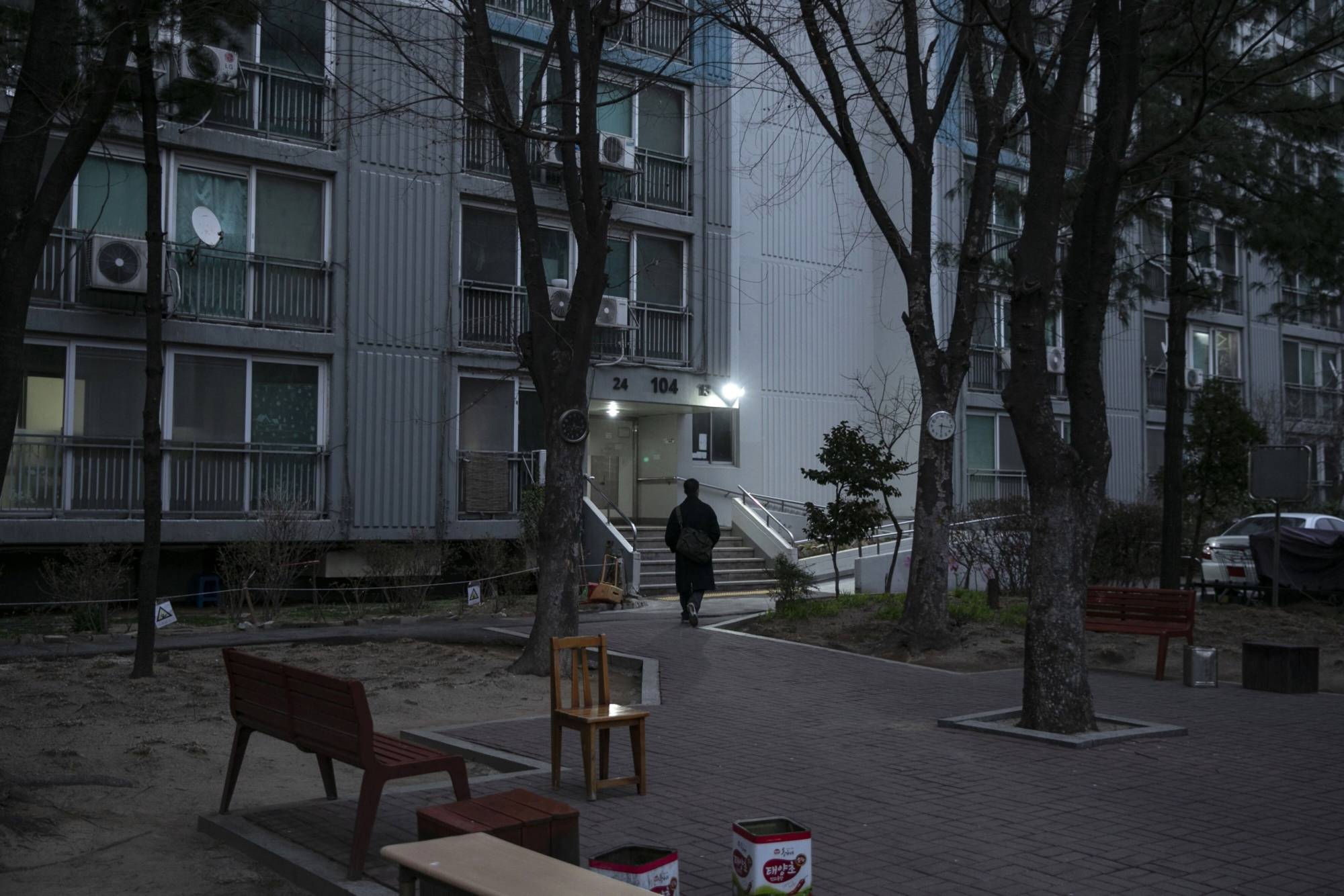The image captures a detailed nighttime scene of a large, white apartment building labelled "26 104," with possibly another number, "15," slightly unclear. Central to the picture is a person in an overcoat, possibly wearing a backpack, climbing a set of six or seven steps toward the entrance of the building. The apartment features multiple windows, some with air conditioning units, and has a balcony with sliding doors. There are two railings flanking the steps. The foreground includes a well-lit walkway leading to the entrance, surrounded by scattered park benches and trees. One bench holds two metal boxes with ads, while another tree has a clock mounted on it. A white car is parked in the middle right of the image, facing away, reinforcing the nocturnal ambiance. The overall scene is clear, vividly capturing the quiet, moody atmosphere of the night.